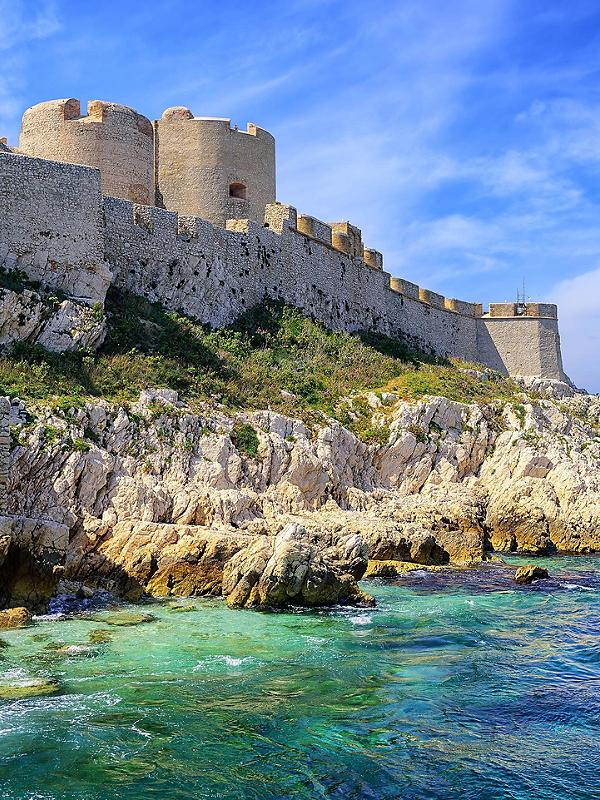The photograph captures a stunning and ancient stone fortress perched on a cliffside overlooking a body of water. The fortress, which evokes imagery of historic edifices like the St. Augustine Fortress in Florida or the Great Wall of China, stands majestically with its beige-gray stone walls and two prominently visible round towers. Above the fortress, the sky stretches out in a vibrant blue, dotted with scattered clouds. The cliff itself is a diverse palette of nature, beginning with patches of green grass leading up to the fortress, and transitioning to an array of rocks in various shades of white and brown. Down below, the cliff descends into clear, light blue water tinged with green hues, which contrasts with the darker waters on the right side of the image. The entire scene is a harmonious blend of natural beauty and historical architecture, creating a captivating and picturesque view.